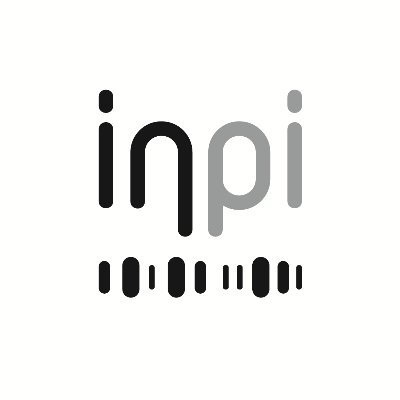The image depicts a minimalist, monochromatic logo on a pure white background. The centerpiece is the text "inpi" rendered entirely in lowercase letters. The letters "i" and "n" are in black, while "p" and the final "i" are in gray. Notably, the 'n' extends downward where it meets the 'p', creating a balanced, aesthetically pleasing design. Directly beneath the text is a line of vertically aligned, pill-shaped ovals in varying sizes, all in black, starting with a larger oval in the center and tapering to smaller ones on either side. The overall style of the logo is sleek and modern, emphasizing simplicity and symmetry.